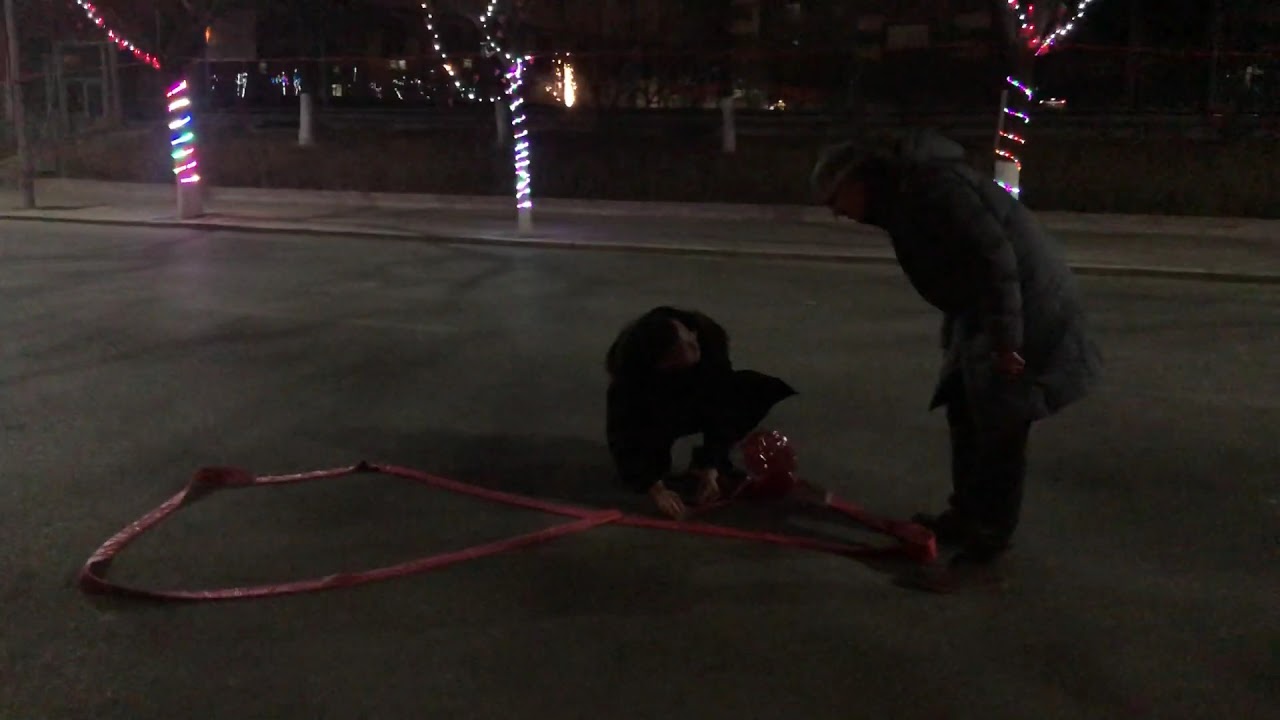The image is taken outdoors at night on a gray asphalt road or walking path, with three trees decorated with colorful Christmas lights spiraling up their trunks. It depicts two people in the center: a man on the right wearing a long gray winter coat and black pants, and another person, possibly a woman, on the left in a black coat. The man is standing with his hands by his side, looking down slightly at the person who is squatting. The squatting individual is manipulating a long red ribbon or bow, shaping it into a circular loop on the ground. In the background, there are additional lights and some buildings visible, suggesting a park or holiday-decorated area. A guardrail and pillars can also be seen in the distance, adding to the nighttime urban atmosphere.